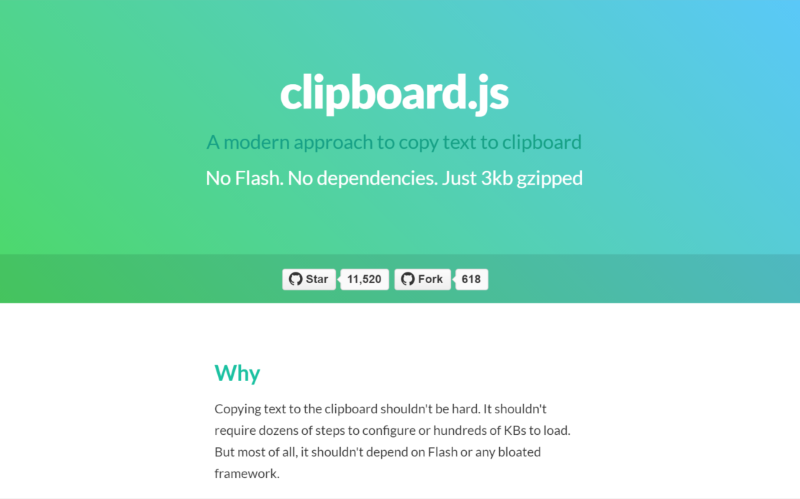This horizontal rectangular image features a gradient background that transitions from a medium-tone green on the left to a combination of blue and turquoise towards the upper right corner. Positioned in the center of the mostly green section, the text "clipboard.js" is written in bold white font, all lowercase and without spaces. Beneath this, in green font, it reads: "a modern approach to copy text to clipboard."

Further down, in white font, it states: "no flash. no dependencies. just 3kb zipped." Below this text, there is a darker horizontal section containing four centered black segments. The first segment features a star icon accompanied by the text "Star" and the number "11,520." The second segment also has a star icon with the text "11,520." Next, is the word "Fork" followed by another icon and the number "618."

Below this, on a crisp white background, the word "Why" is written in green font. The subsequent black text reads: "Copying text to the clipboard shouldn't be hard. It shouldn't require dozens of steps to configure or hundreds of KBs to load. But most of all, it shouldn't depend on flash or any bloated framework."